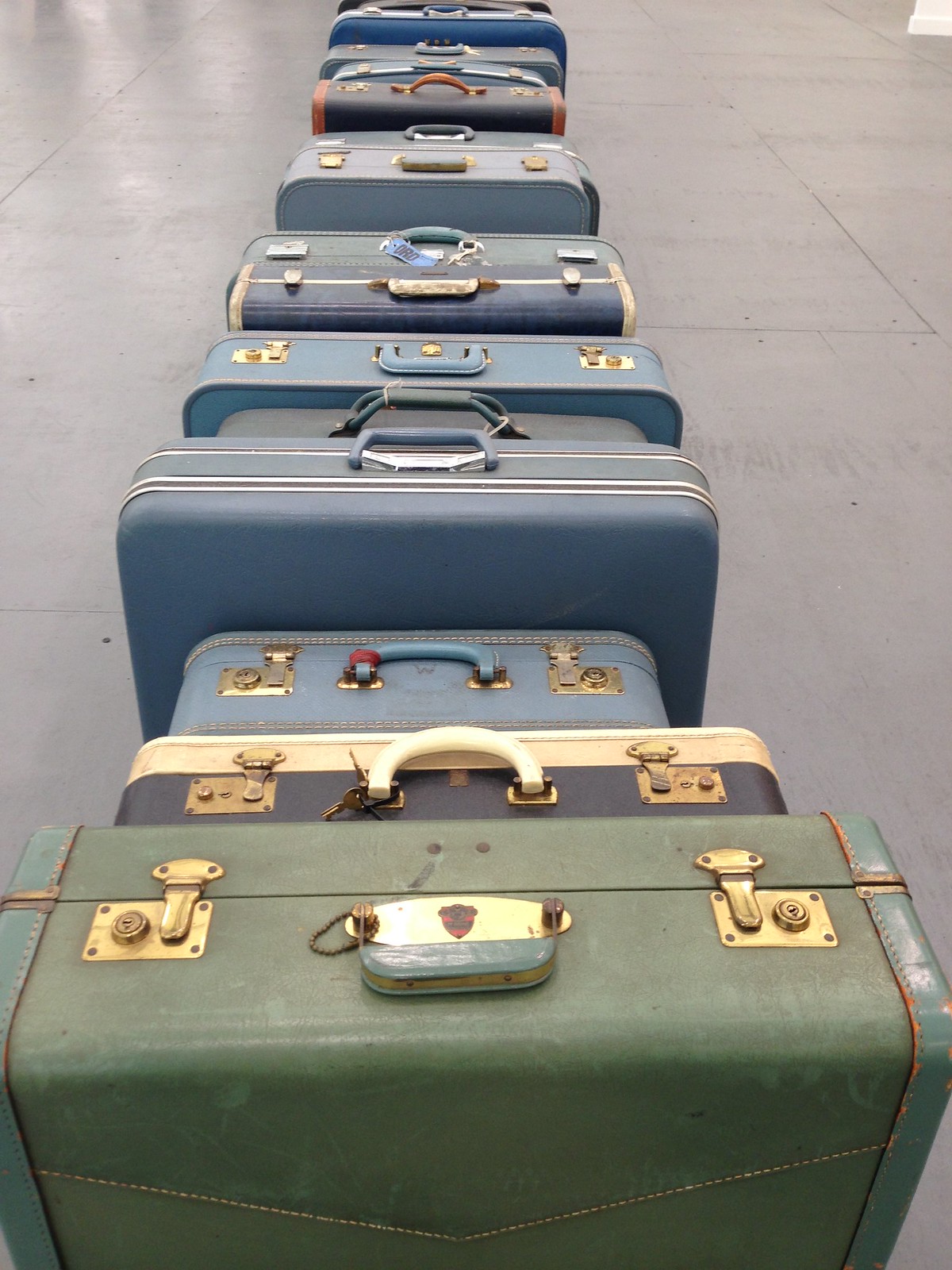The photograph showcases a striking row of vintage suitcases lined up vertically, viewed in profile with the bottom sides facing the camera. Set against a pristine white background reminiscent of large ceramic floor tiles, the suitcases gradually diminish in size as they extend from the bottom to the top of the image, creating a cascading visual effect. The prominent, largest suitcase at the forefront is a vibrant green with gold locks and latches. Adjacent to it is a smaller, predominantly brown and tan suitcase. Beyond these, a series of blue suitcases in various sizes, including an attaché case, are noticeable, with one of them displaying dark blue with orange accents. In the distance, a black attaché-style suitcase edged in brown caps off the collection. The suitcases feature round handles fixed with metals of varying finishes—gold, brass, and silver—enhancing their vintage charm. The arrangement of these suitcases, resembling a line of dominoes, emphasizes the nostalgic aesthetic of classic travel accessories with functional latches and lockable designs.